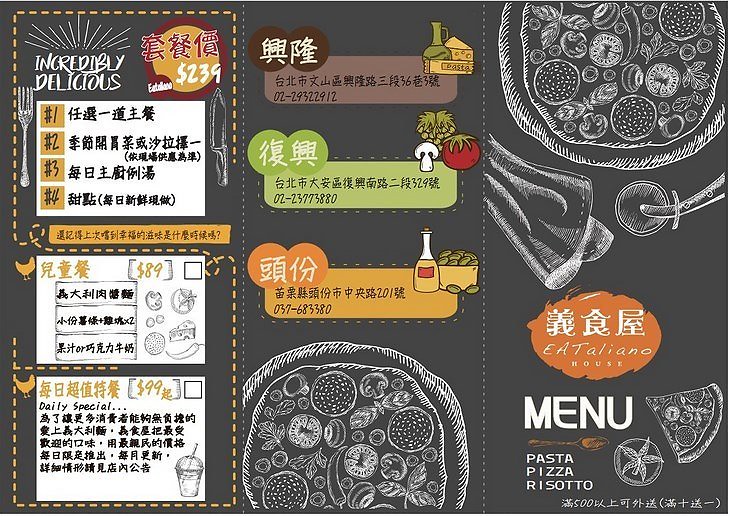The image depicts a visually striking menu with a black background, primarily in an Asian language, possibly Chinese, interspersed with English text. The menu is divided into three vertical sections, each richly decorated with food illustrations and text.

In the far-right section, the heading reads "Menu" in English at the bottom right corner. Underneath this, English text lists the words "pasta," "pizza," and "risotto." Adjacent to this, there is a visual icon featuring a slice of pizza and a herb surrounded by a circle. Toward the top, additional food imagery includes red sticks, a dipping cup, and a bowl filled with various ingredients. Above all, this section prominently displays "EAT T-aliano House" in stylized capital and lowercase letters.

The central section highlights three small text bubbles, each with different food illustrations and text, color-coded as brown, green, and orange. The brown bubble shows cheese and wine, the green one features mushrooms, tomatoes, and grapes, and the orange bubble depicts olives or similar items. Below these, another bowl of herbs is illustrated.

The left section begins with the phrase "Incredibly Delicious" in English, followed by a list of four menu specials, numbered one through four. Accompanying these specials are images, including pork and other appetizers, with their respective prices shown in Asian characters, likely denoting some local currency such as pesos or sen. Towards the bottom, this section also includes the text "Daily Special" in English alongside a beverage listing priced at $99 in gold writing.

Collectively, the menu is a fusion of Italian and Asian culinary elements, reflecting the name "EAT T-aliano House". A coherent blend of detailed foo imagery and the juxtaposition of English and Asian text makes it clear that this menu is crafted for an Italian restaurant operating within an Asian linguistic and cultural context.